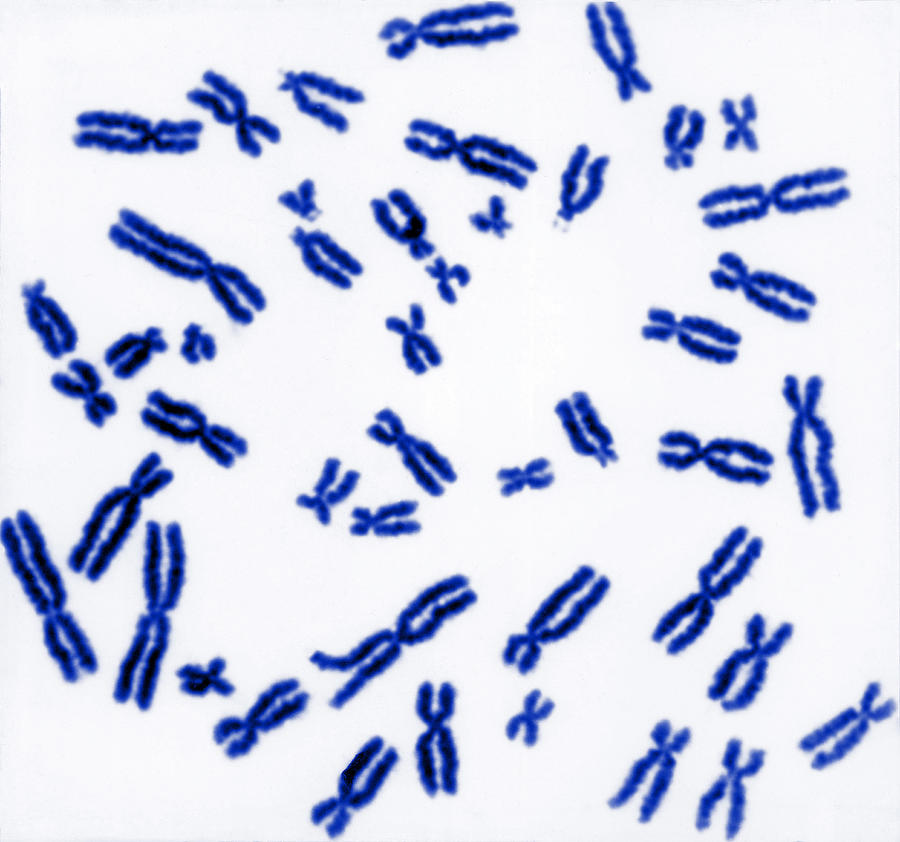This is a highly detailed, color-enhanced microscopic photograph showcasing approximately 30 to 35 chromosomes, meticulously stained in varying shades of blue to highlight their intricate structures against a predominantly white background with a slight off-white, light gray tint. Each chromosome is presented in a characteristic slightly compressed X shape, resembling bow ties, and they are scattered unevenly across the image. The chromosomes, which vary in length with some appearing notably longer or shorter than others, are predominantly situated around the perimeter of the square frame, with more white space centralized, drawing the observer’s gaze outward. Upon closer examination, some chromosomes appear darker in the center, almost black, framed by the blue stain, giving them a three-dimensional, textured look. The image displays no text or additional markings, focusing entirely on the natural form and diversity of the chromosomes themselves.